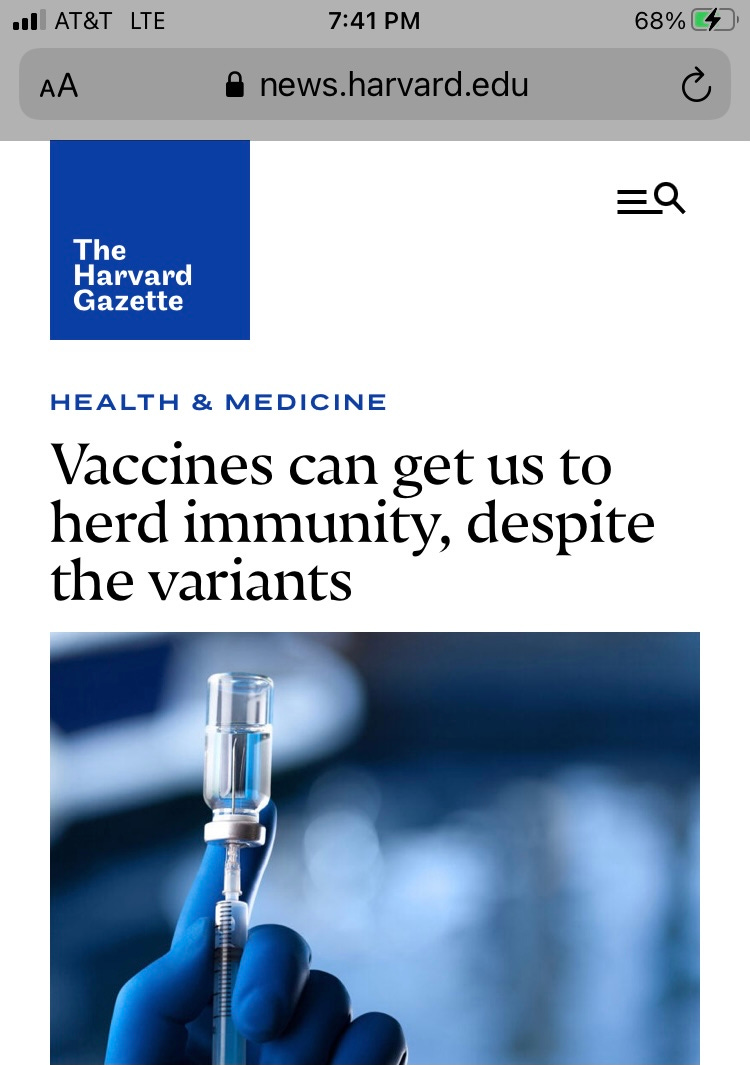In this detailed screenshot from a smartphone, you can see various interface elements and a webpage. At the top, there's a gray status bar indicating three bars of AT&T LTE service, the time as 7:41 PM, and a battery life of 68%. 

Directly below the status bar is an address bar displaying "news.harvard.edu," leading to the Harvard Gazette's webpage.

The webpage itself has a white background. In the top left corner, there's a dark blue square with the text "Harvard Gazette" in small white letters. The top right corner features three black lines, representing a menu icon, and a magnifying glass, suggesting a search function.

Highlighted in blue text on the white background are the words "Health & Medicine," indicating the content category. Below, in black text, is the article title: "Vaccines can get us to herd immunity despite the variants."

Under the title is a horizontal rectangular image depicting a medical scene. A person's hand, covered by a blue latex glove, is holding a clear glass vial filled with liquid. The person is drawing some of the liquid into a hypodermic needle from the vial. The background of this image is a distinct blue, complementing the professional and informative nature of the webpage.